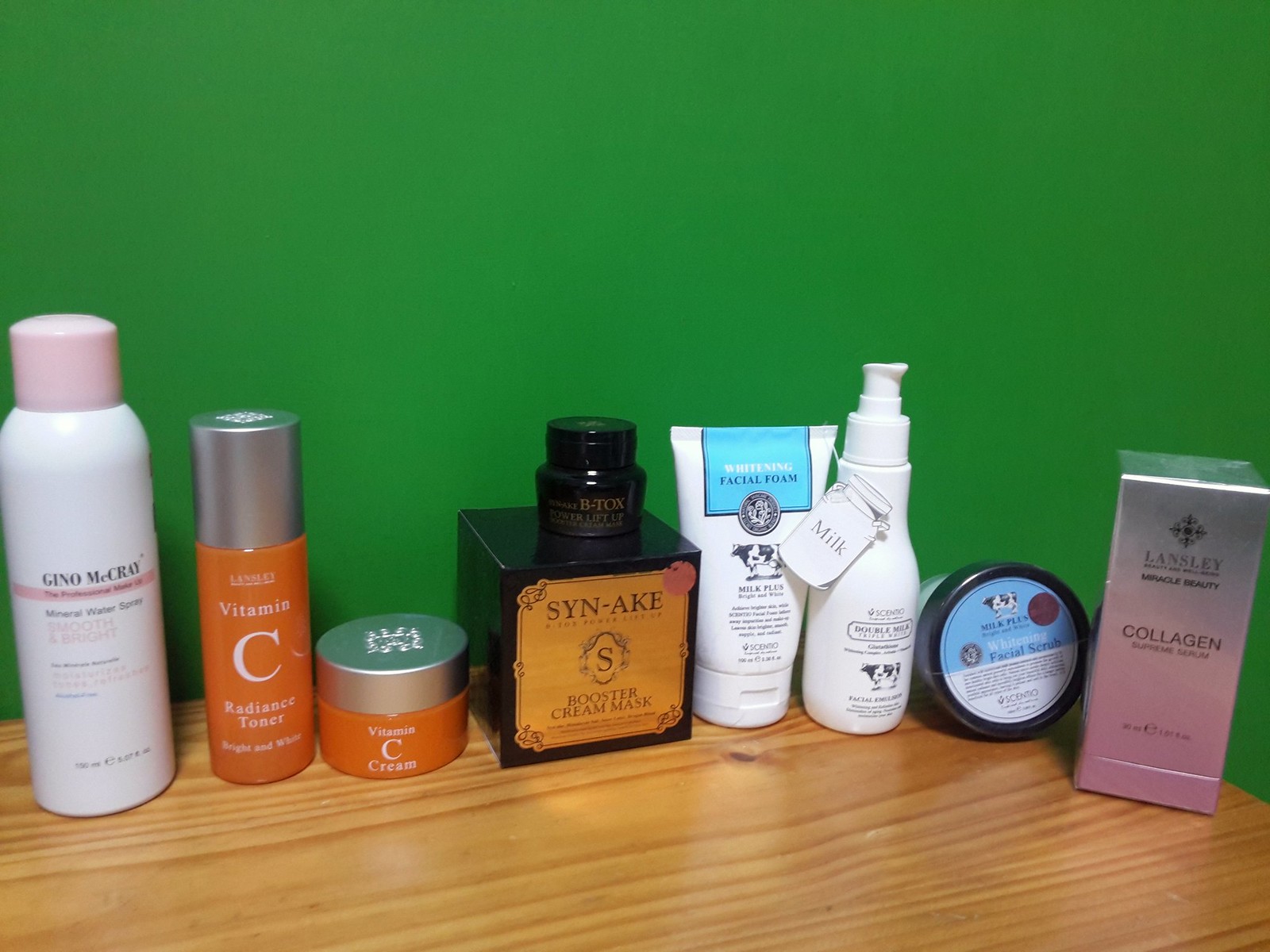This realistic photo captures a short, rounded wooden table with visible wood grain and a notable dark burn mark. Behind the table, the wall is painted solid dark green. The tabletop features an array of beauty products neatly lined up with labels facing the camera. 

From left to right: 

1. A white bottle with a pink lid, bearing faint black writing, which includes the name "Gino McRae."
2. An orange bottle with a silver lid labeled "Vitamin C" in white writing.
3. Another orange bottle of the same smaller size and silver lid, labeled "Vitamin C Cream."
4. A black square bottle with a tan label that reads "Sanake" and features a stylized 'S.'
5. Two white bottles, one of which has a squirt top and depicts a cow with a label saying "Milk."
6. A small black dish with a blue lid.
7. Lastly, a silver and pink box labeled "Collagen."

The details of the items and the contrasting background create an aesthetically pleasing and organized composition.